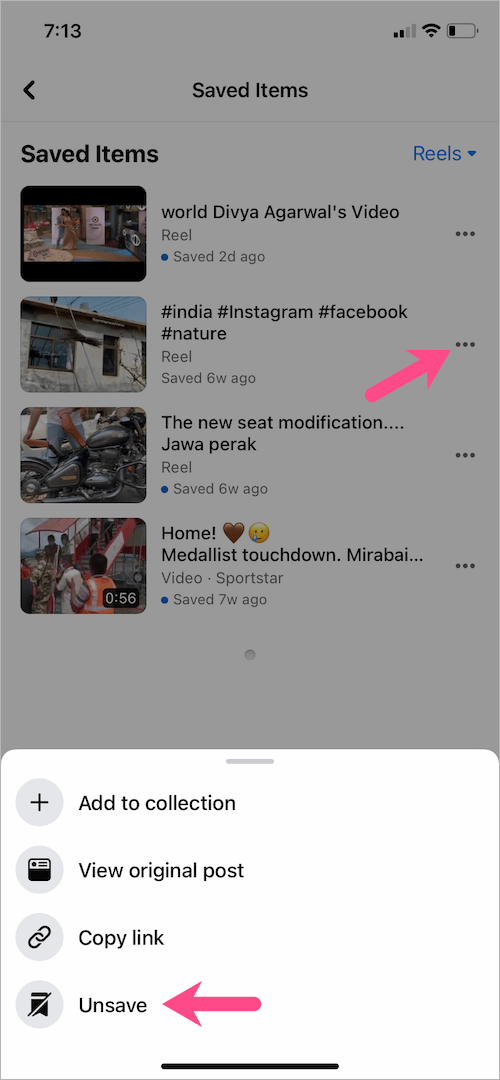**Detailed Caption:**

The image depicts a section from the Instagram Reels interface, specifically the "Saved Items" page. The top two-thirds of the image feature a gray background that serves to indicate the interface background details. At the very top left corner, the time is displayed as "7:13," followed by two bars of cellular signal, full WiFi connectivity, and a battery icon showing approximately 20% charge remaining.

Below this top bar, the interface includes a back button on the left with the label "Saved Items" in black text. Adjacent to this, on the right side, the word "Reels" appears in blue with a downward arrow indicating a dropdown menu.

The content begins with a section labeled "World Devia's Video Reel," saved two days ago. Below this first entry are several hashtags: #India, #Instagram, #Facebook, and #Nature.

Further down, another entry shows "Reel saved six weeks ago," featuring a red arrow pointing to a hamburger menu icon on the right side of this entry.

The next saved item is titled "The New Seat Modification, Jawa Perak," also saved six weeks ago. Following this is another reel titled "Home" illustrated with a brown heart emoji and a crying emoji, concerning Medalist Touchdown Mirabai, saved seven weeks ago.

Below these items, from a submenu of the "Hashtag India" section, the image shows options such as "Add to Collection," "View Original Post," "Copy Link," and "Unsave" with respective icons on the left. A red arrow highlights the "Unsave" option.

The detailed layout helps to distinguish each saved reel and various interface elements, clearly showing the organization and categories within the Instagram Reels "Saved Items" page.